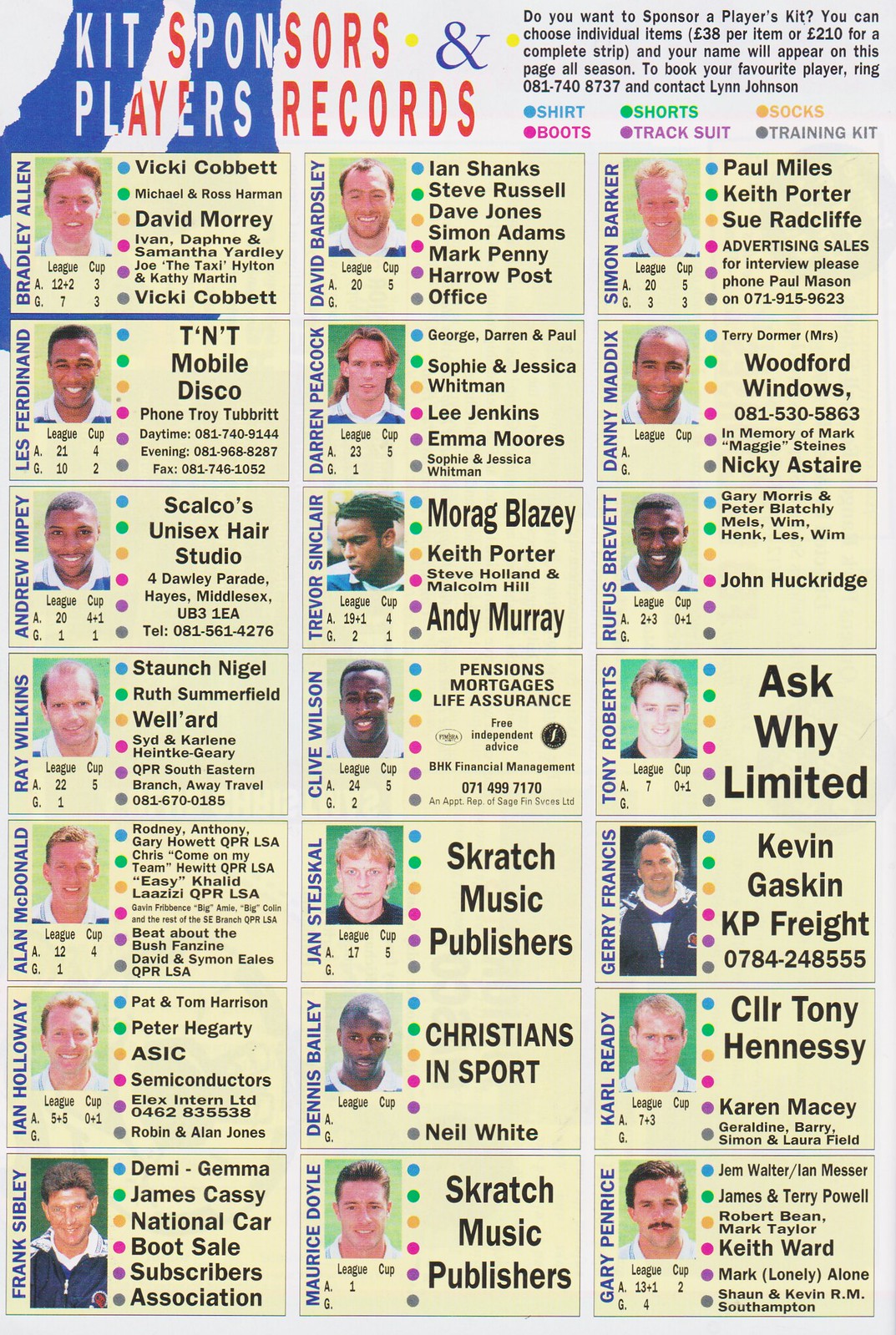The image is a detailed grid featuring columns and rows of football players' faces alongside their sponsorship information. At the top, a header against a blue and white background reads, "Kit Sponsors and Players' Records." Adjacent to this, an informational section asks, "Do you want to sponsor a player's kit? You can choose individual items for £38 each or £210 for a complete strip, and your name will appear on this page all season. To book your favorite player, ring 081-740-8737 and contact Lynn Johnson." Below, players are organized in yellow boxes, each containing a player's photo with their name running vertically in blue on the left side. Each box also features colored dots corresponding to different kit items: blue for shirts, green for shorts, orange for socks, pink for boots, purple for tracksuits, and gray for training kits. Names of sponsors like Vicki Cobbett and Joe the Taxi Hilton are listed below the player's photo. The image showcases multiple columns and rows with detailed sponsorship information, emphasizing the opportunity for fans to support their favorite footballers.